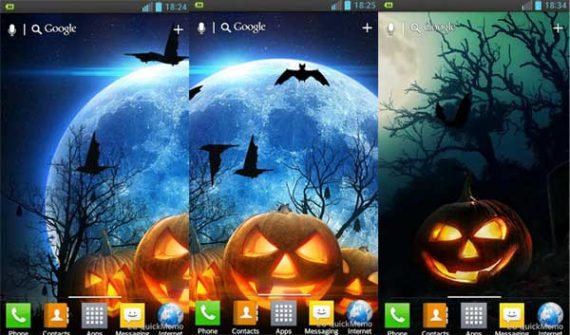A series of three phone screen wallpapers are displayed side by side, each depicting a Halloween-themed night sky. 

**First Wallpaper (Left):**
- **Theme:** The scene captures a spooky night.
- **Details:**
  - **Moon:** Crescent moon positioned at the left.
  - **Bats:** Two bats are flying in front of the moon.
  - **Tree:** A gnarled tree on the left side with two bats hanging from its branches.
  - **Jack-o'-lanterns:** Positioned at the bottom right, one and a half jack-o'-lanterns are visible, with the one on the left closer to the viewer.
  - **Phone UI Elements:** 
    - A green battery icon on the top left.
    - A signal strength indicator (3 out of 5 bars) on the top right next to a blue box reading "1824".
    - The bottom of the screen features icons for phone, contacts, apps, messaging, quick memo, and internet.
    - A plus symbol, a microphone icon, a separator line, a search icon, and the word "Google" are situated in the top left corner.

**Second Wallpaper (Middle):**
- **Theme:** Continuation of the moonlit Halloween night.
- **Details:**
  - **Moon:** Full moon centered with bats flying around.
  - **Bats:** Three full bats and the right wing of a fourth bat are visible.
  - **Jack-o'-lanterns:** Three jack-o'-lanterns at the bottom, with the middle one's face fully visible and the other two partially obscured.
  - **Tree:** Bare tree branches silhouette against the glowing moon.
  - **Phone UI Elements:** 
    - Battery, signal strength, and other UI components are similar to the first wallpaper.
    - The time has updated to "1825".

**Third Wallpaper (Right):**
- **Theme:** A darker, greener Halloween night.
- **Details:**
  - **Moon:** The moon is not prominent, casting a darker greenish hue over the scene.
  - **Bats:** One bat is flying amidst the trees.
  - **Tree:** More of the tree is visible, adding to the eerie atmosphere.
  - **Jack-o'-lantern:** A single large jack-o'-lantern is centered at the bottom.
  - **Phone UI Elements:**
    - Identical layout to the first two wallpapers with a slight change in details like the time updated to "1834".

Overall, each wallpaper embodies a unique and spooky Halloween theme with consistent phone UI elements, changing the moon phases, bats, trees, and jack-o'-lantern arrangements.